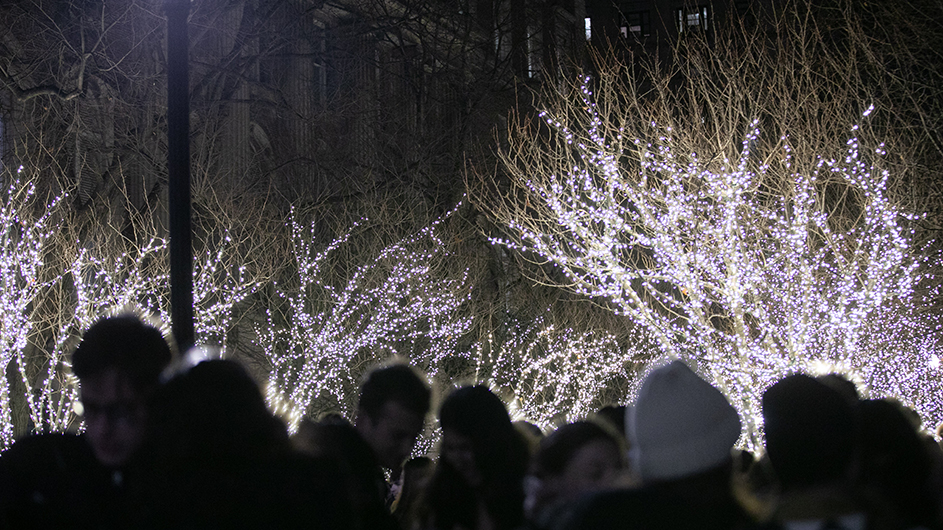In this nighttime photograph, a group of mostly Caucasian men and women gather in the chilly outdoor setting, dressed in winter attire. Predominantly, a man wearing a white beanie stands out among the crowd, which is positioned at the bottom of the frame and appears slightly out of focus. The people are engaged with each other or their phones, including a noteworthy couple— a woman with long dark hair and a man with short light hair— sharing an object in their hands. Behind them, barren trees adorned with brilliant, clear white lights suggest a festive, holiday season atmosphere, like Christmas. These illuminated trees draw the main focus of the image and stretch across both sides and through the center, leaving some small branches unlit. Further back, just barely recognizable, are several old-style buildings, partially hidden by the trees and adorned columns. One tall building is particularly notable, with some windows lit, extending out of the frame. Near the left side, there's also a lantern pole visible, adding to the wintry, festive scene.